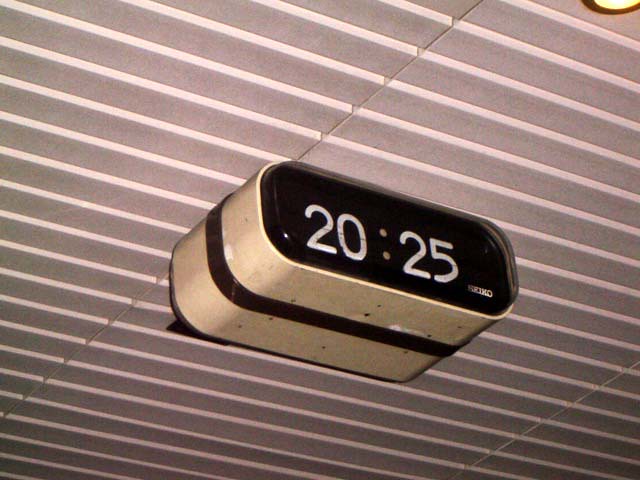In this rectangular image, we observe a ceiling comprised of white slats extending uniformly across the frame. Suspended from the ceiling is an oblong, vintage Seiko clock, which appears to be securely mounted and slightly aged. The clock features a white metal exterior and a contrasting black band encircling its center. The digital screen on the clock's lower right displays bold white numbers reading "2025." In the upper right corner of the image, a faint glow emanates from a recessed light fixture that is turned on, adding a hint of illumination to the scene. The perspective of the photo captures the underside and left side of the clock, showcasing its attachment to the ceiling and highlighting its retro design.